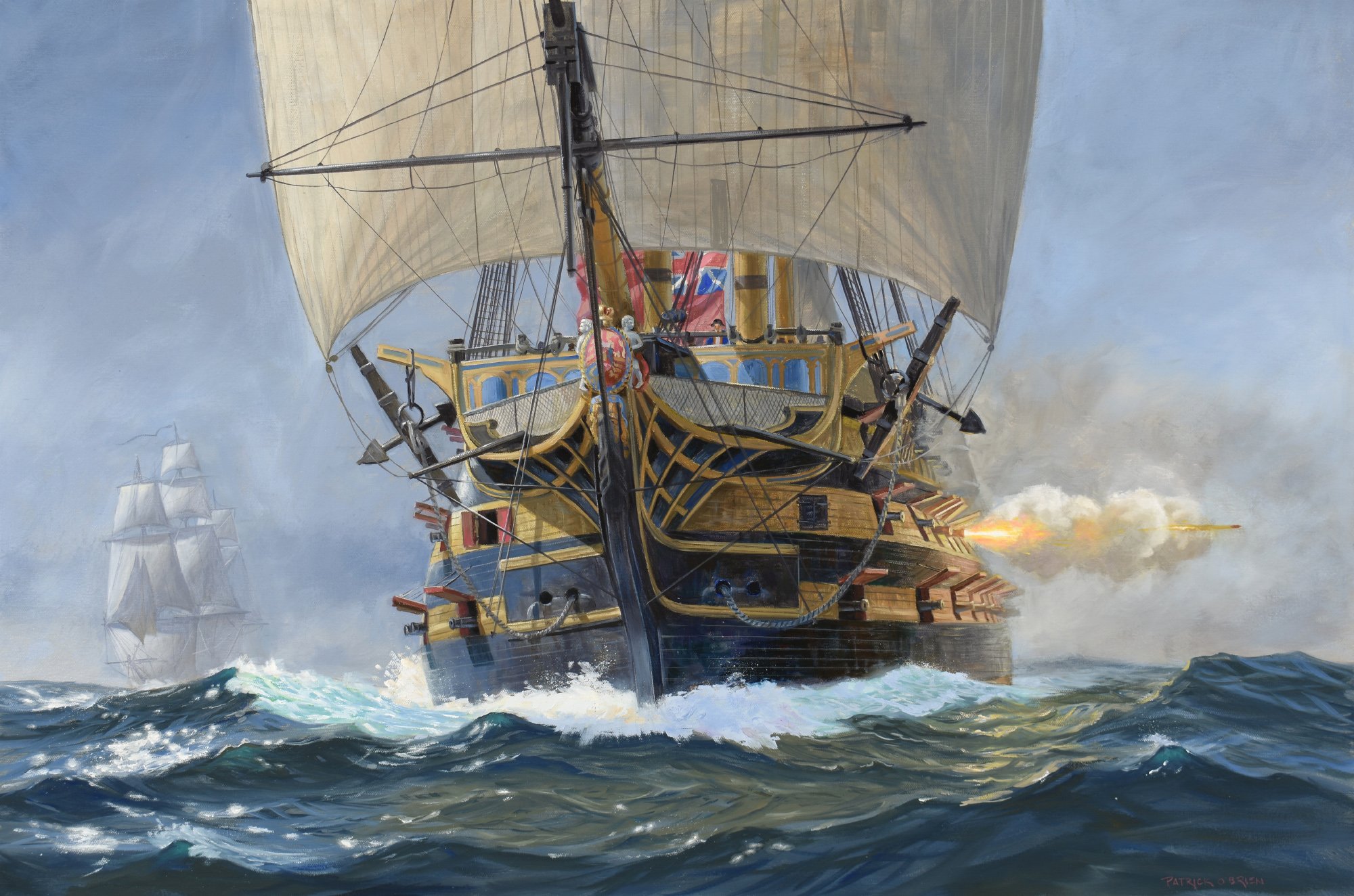This detailed painting depicts a large, old-fashioned pirate ship navigating through a choppy, dark-blue ocean. The viewer's perspective is from the front, looking directly at the ship with its wooden sides and distinctive yellow and black siding. The ship boasts three visible levels, each lined with open cannon doors, and many cannons are protruding. On the top right side, a bright yellow-white flame and clouds of white and dark smoke mark the firing of one cannon, its projectile seen streaking away. The ship is well-rigged, with numerous rope lines, and features a large sail at the bow, billowing forward in the wind. Anchors are visible on both the left and right sides of the ship. In the background, another ship with furled sails appears on the left, adding to the scene’s dynamic intensity. The sky is a contrasting light blue, enhancing the realism and old-fashioned charm of the painting.